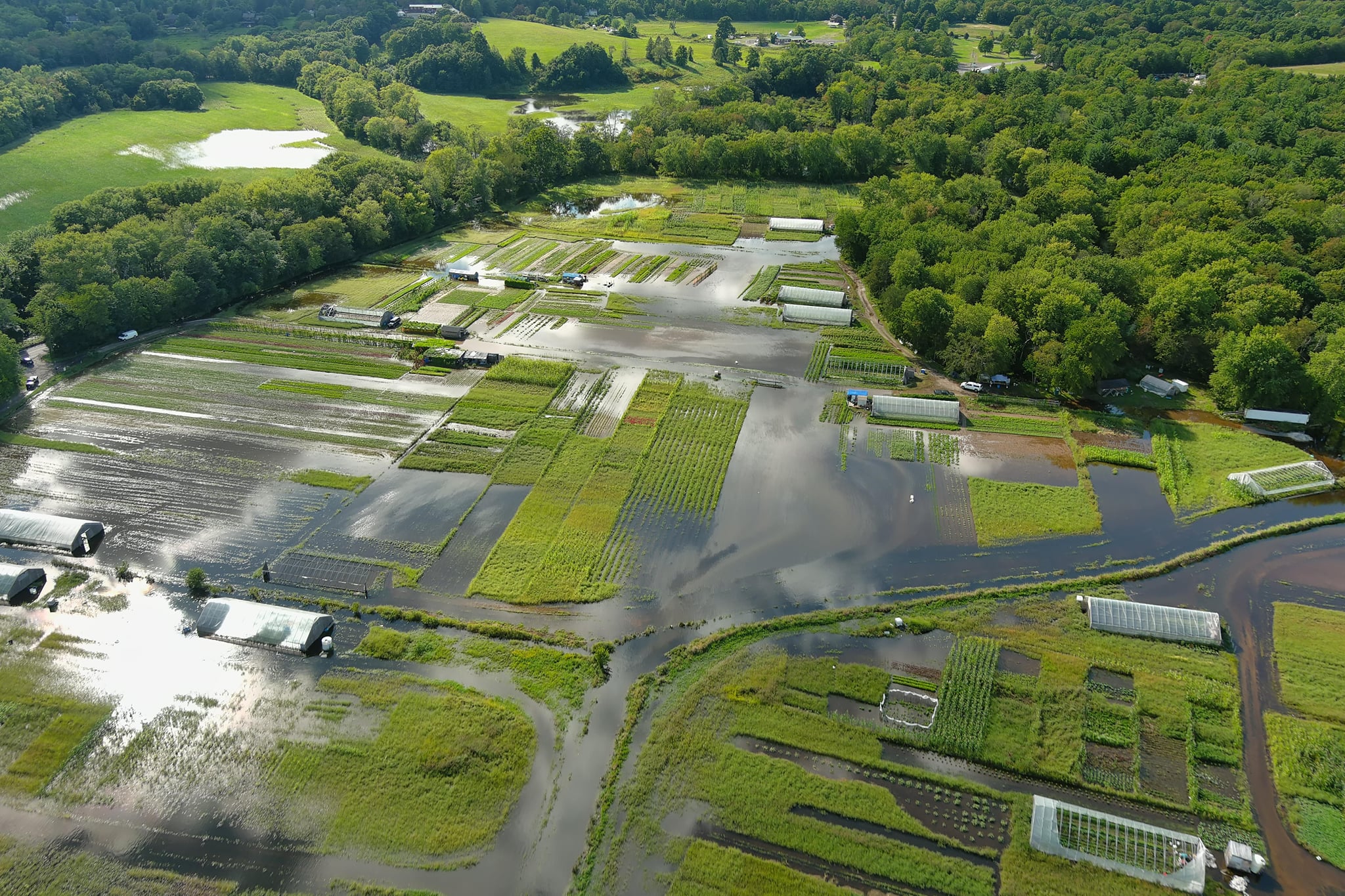This image is an aerial shot likely taken by a drone, showcasing a flooded farmland. The foreground is dominated by submerged fields with rows of crops intermittently visible above the water's surface. Amidst the farm area, there are about ten long structures resembling greenhouses, some with transparent roofs and others covered in white canopies, particularly noticeable towards the lower left side of the image. The central and bottom portions of the farm appear extensively flooded, with water creating a patchwork of submerged and elevated land areas. The background features a dense lining of lush, green trees, especially prominent to the top right, transitioning to more sporadically placed trees and additional farmland towards the top left. Distant farmhouses are also discernible in the background, adding a human element to the otherwise waterlogged landscape.